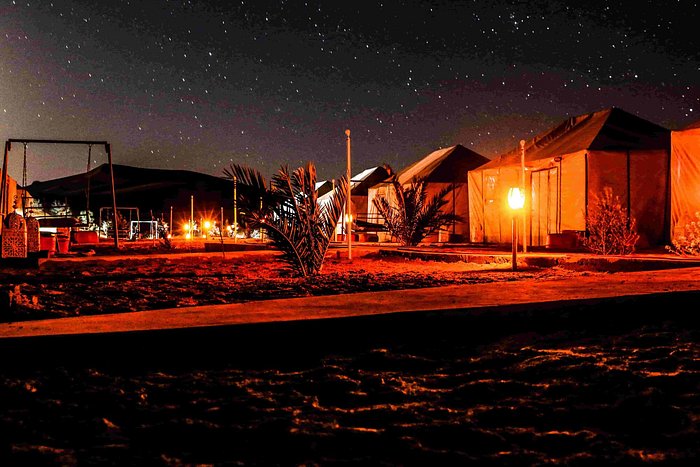The image is a nighttime landscape with a distinct reddish hue, possibly due to a filter applied to the photograph or painting. It depicts a campground featuring large, house-like tents on the right side and a training or playground area in the foreground. The ground is dotted with white poles, and in the background, dark mountains loom under a very dark sky filled with an abundance of stars. Scattered lights and various types of recreational equipment, including what looks like swing sets, add to the scene’s ambiance. The overall setting exudes a blend of tranquility and adventure, bathed in a surreal, red-tinted glow.